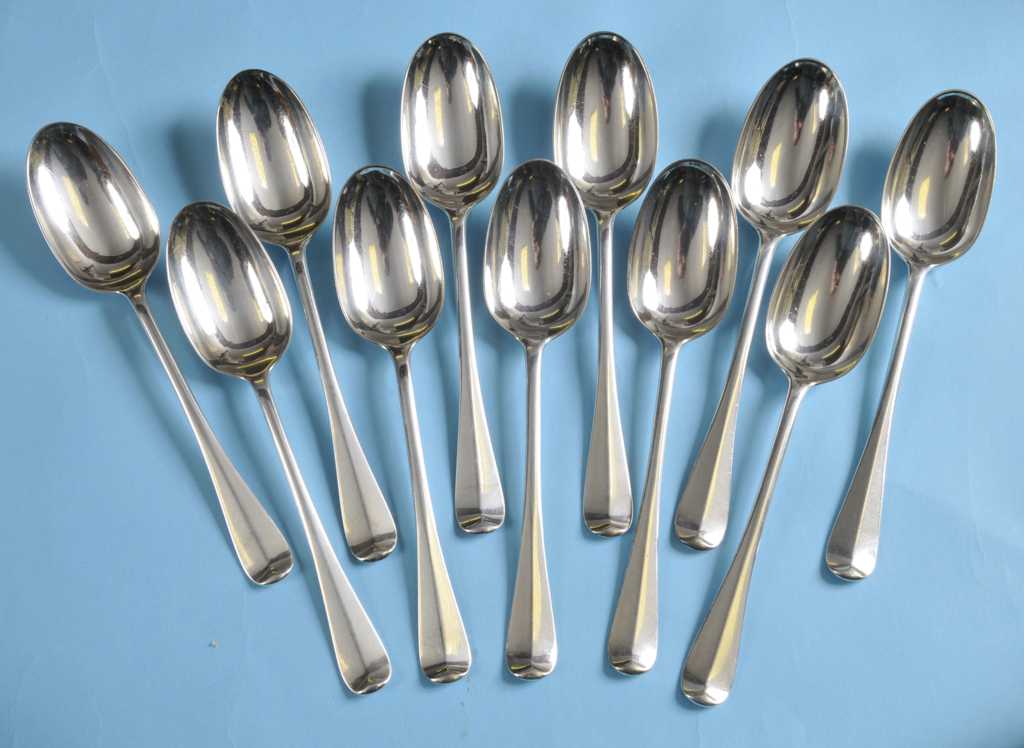The image features an elegantly arranged set of 11 silver spoons, meticulously positioned against a sky-blue background that enhances their reflective, polished surfaces. The spoons are displayed in two rows, with six spoons in the top row and five in the bottom row, placed in between the spoons above. The arrangement creates a visually appealing pattern, almost resembling a fan or a semicircle, with the handles of the spoons tilting slightly outward. This professional, minimalist photograph highlights the sleek, long-stemmed design of the spoons, showcasing their sophisticated and high-quality appearance. No text or signage distracts from the simplicity and beauty of the silverware and the serene blue backdrop.